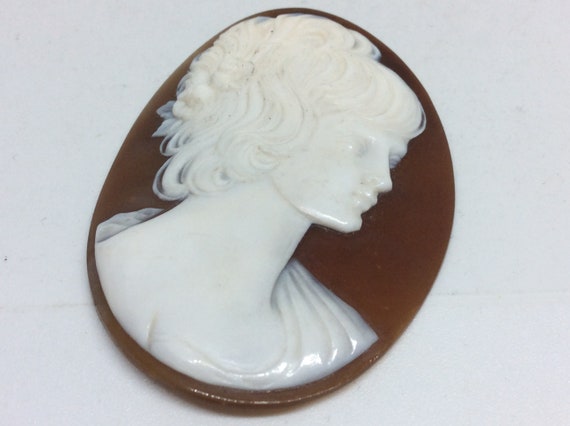The image features a Greco-Roman artifact, an oval-shaped ornament of chocolate brown color resting on a pale, grayish-white background. The focal point of the piece is a meticulously carved profile of a head, depicted in a cream or white material, standing out strikingly against the brown base. The profile appears to be that of a figure from early centuries AD, rendered with precise details including a square chin, carved eyes, a defined nose, and short curly hair styled in an updo with bangs towards the eyebrows, evoking a Roman or Greek aesthetic. The figure's attire shows the draped fabric characteristic of a Roman toga, with visible grooves and indentations enhancing the realism of the carving. The head, neck, and hair of the portrait are distinctly white, providing a sharp contrast to the brown, flat oval surface. The artifact is viewed from an angled perspective, as if from above, highlighting the depth and engraving work of the piece.